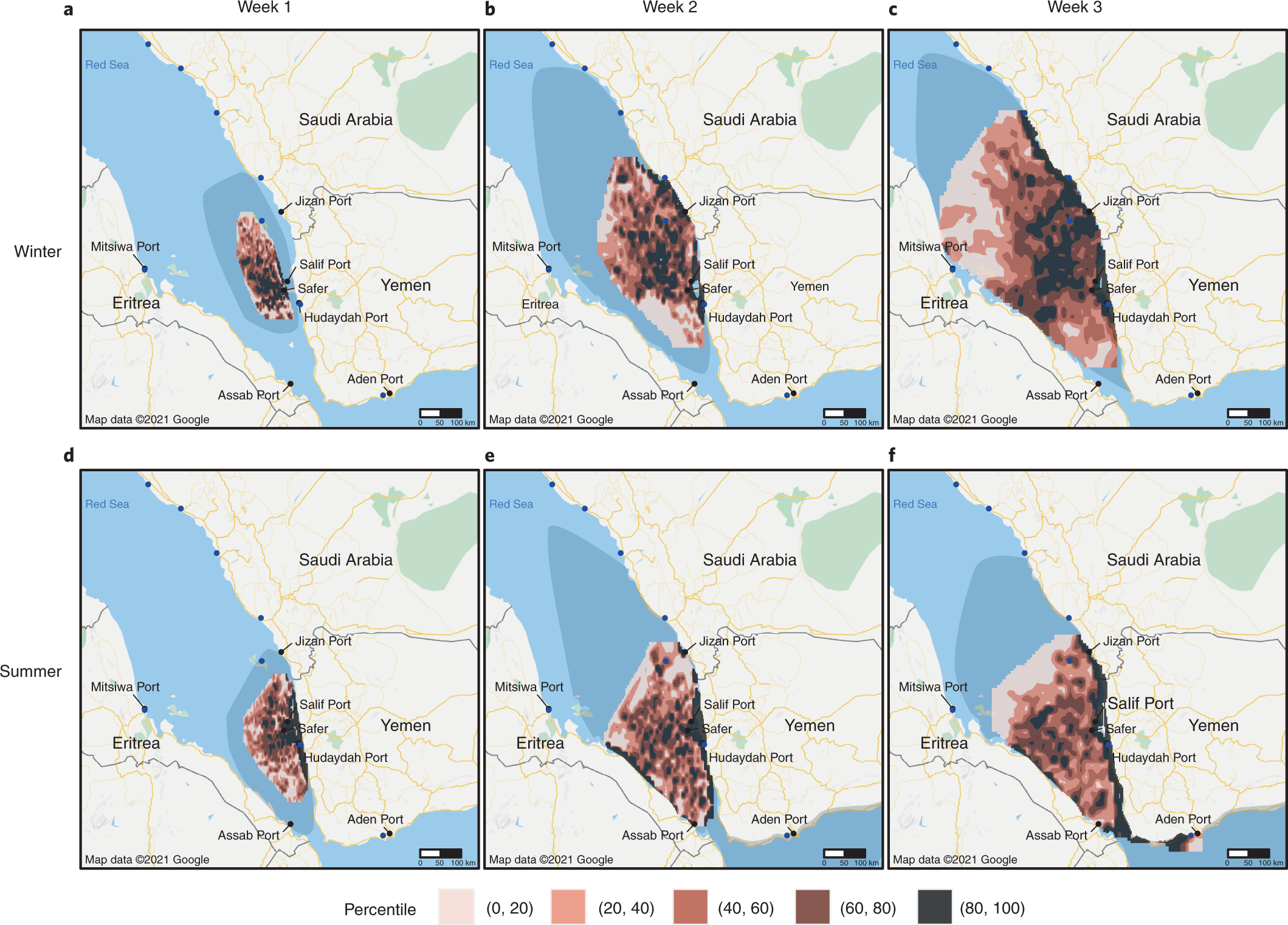The image is a color diagram consisting of six maps organized in two rows. The top row represents winter, with maps labeled Week 1, Week 2, and Week 3. The bottom row depicts summer with similarly labeled weeks. Each map showcases regions including Saudi Arabia, Yemen, and parts of the Red Sea, with a color-coded percentile legend below.

In the winter row, Week 1 depicts a small blob of coloration off the coasts of Yemen and Saudi Arabia. This blob indicates percentages ranging from 20 to 100, with darker colors showing higher percentiles. By Week 2, the blob has significantly expanded, covering more than half the sea area between the countries, primarily in the 40 to 100 percentile range. By Week 3, the entire Red Sea between Saudi Arabia and Yemen is covered, with the darkest colors (80 to 100 percentile) dominating the coastal regions.

In the summer row, Week 1 displays a smaller blob confined to the Yemen side, primarily in the 40 to 100 percentile range. By Week 2, the blob extends across the sea to the coast of Eritrea. The 80 to 100 percent range spreads along the edges, with lower percentiles farther out into the sea. By Week 3, the map shows 80 to 100 percent coverage along the coasts of both Yemen and Eritrea, with the central sea area filled predominantly by 60 to 80 percent.

The percentile key at the bottom of the image uses a gradient from light brown (0-20 percent) to black (80-100 percent), helping to interpret the varying intensities depicted in the maps.